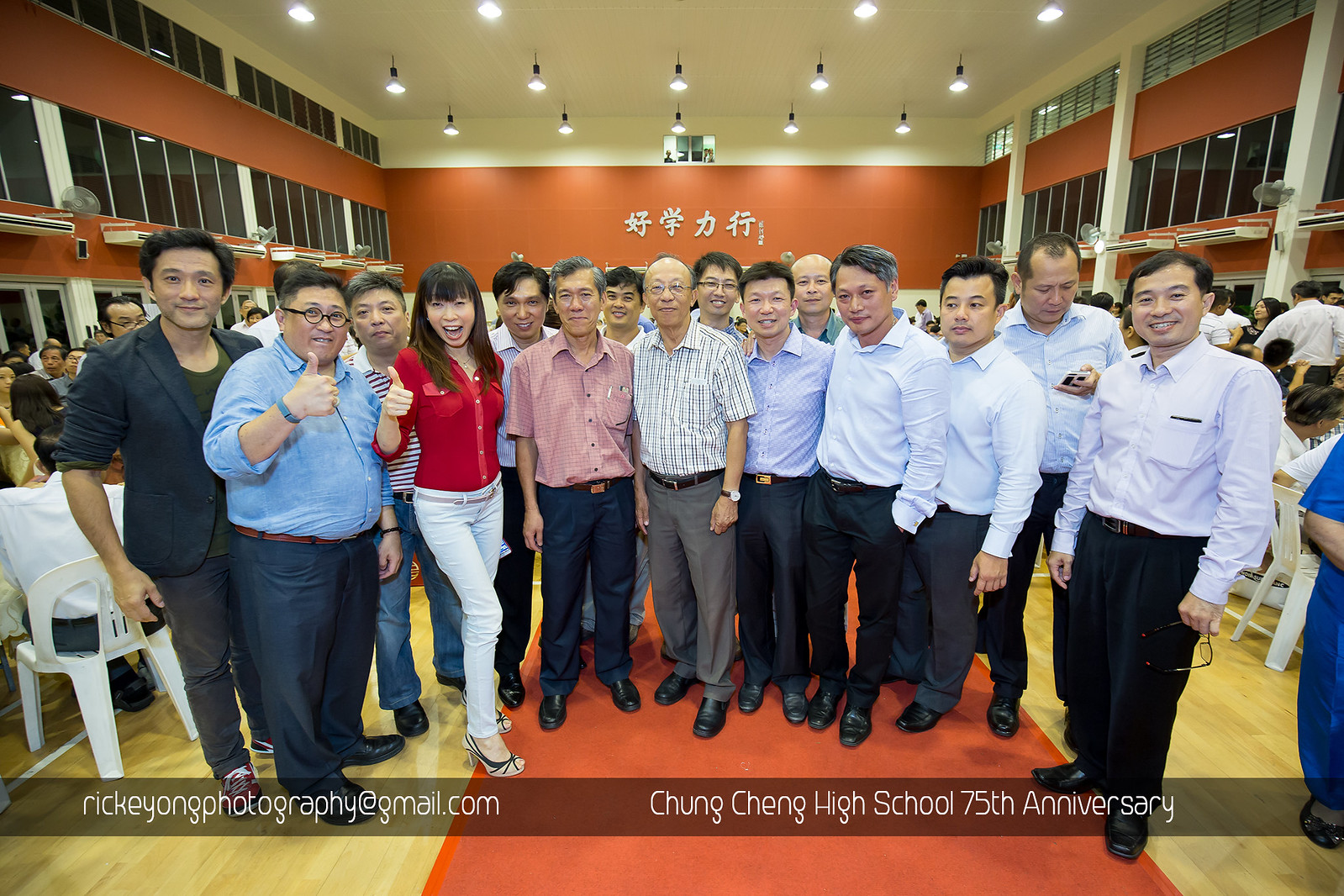In this vibrant scene, a large group of predominantly Asian individuals stands relaxed and smiling in a spacious room. The group, primarily composed of men donning blue collared shirts and slacks, is diverse in age and dress. One notable figure is a very pretty young woman with long black hair, dressed in a striking red top, white pants, and high heels, seated on a simple white plastic chair towards the front.

The backdrop features an orange-brown wall embellished with Asian symbols, beneath a cream ceiling with fluorescent lights. The floor is a blend of wood and an orange center section, adding warmth to the scene. Framing the image is a prominent transparent strip across the bottom bearing the text "rickeyongphotography@gmail.com" and "Chung Cheng High School 75th Anniversary" in white print. The colors in the image are a harmonious mix of black, white, gray, orange, brown, yellow, pink, silver, and blue, complementing the cheerful and celebratory atmosphere of this high school reunion.